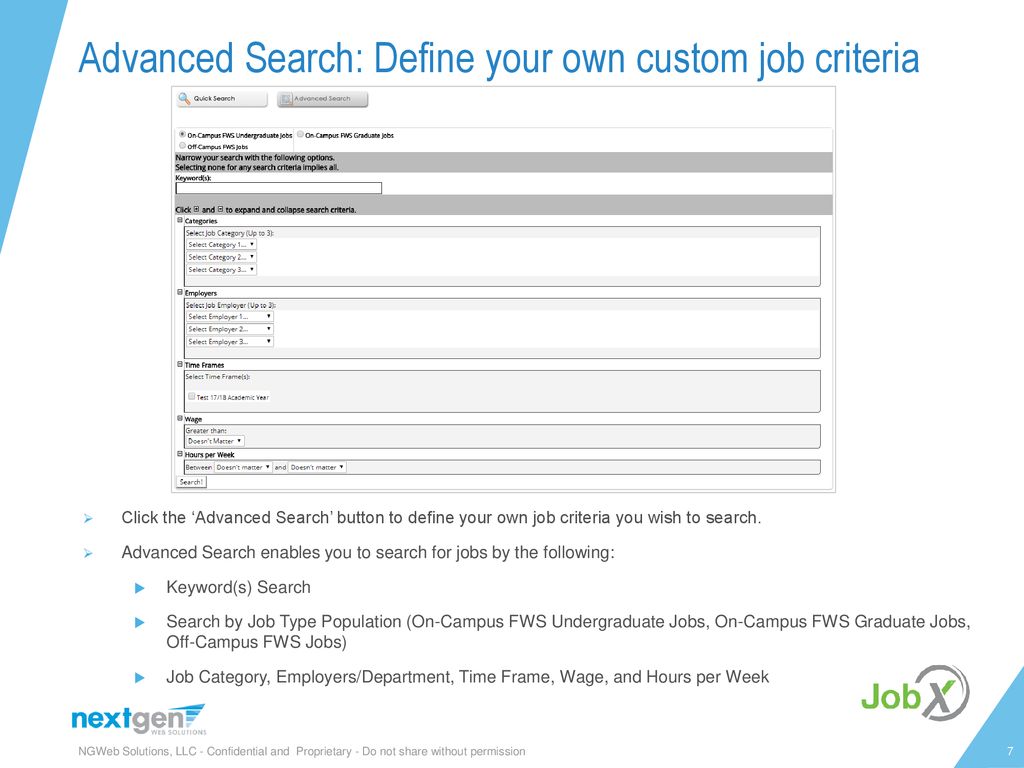The image is a detailed interface for an advanced job search tool. At the top, there is the heading "Advanced Search: Assign Your Own Custom Job Criteria" written in blue, accompanied by a blue upside-down triangle. The majority of the background is white. Beneath the heading, a central gray and white box contains multiple smaller boxes, lines, and drop-down menus. The text within this box is quite small and dark, making it hard to read. 

At the top of the gray and white box, there appears to be a search icon followed by various sections marked by dark writing on a dark gray background. These sections include blank boxes and several more drop-down menus and items. However, the details of these sections remain unclear due to the small and dark print.

Below this main content area, on the plain white background, instructions read: "Click the 'Advanced Search' button to define your job criteria you wish to search." Further details specify that the advanced search enables users to filter jobs by keyword, job title, population (with options such as on-campus FWS undergraduate jobs, on-campus FWS graduate jobs, off-campus FWS graduate jobs), job category, employers, department, time frame, wage, and hours per week. Each of these criteria is marked with a blue triangle.

At the bottom of the image to the left, the text "Next Gen" is displayed in blue and gray. In the far right corner, "Job X" is written in green and gray, accompanied by a final blue triangle. The copyright information is also located at the bottom, near "Next Gen".